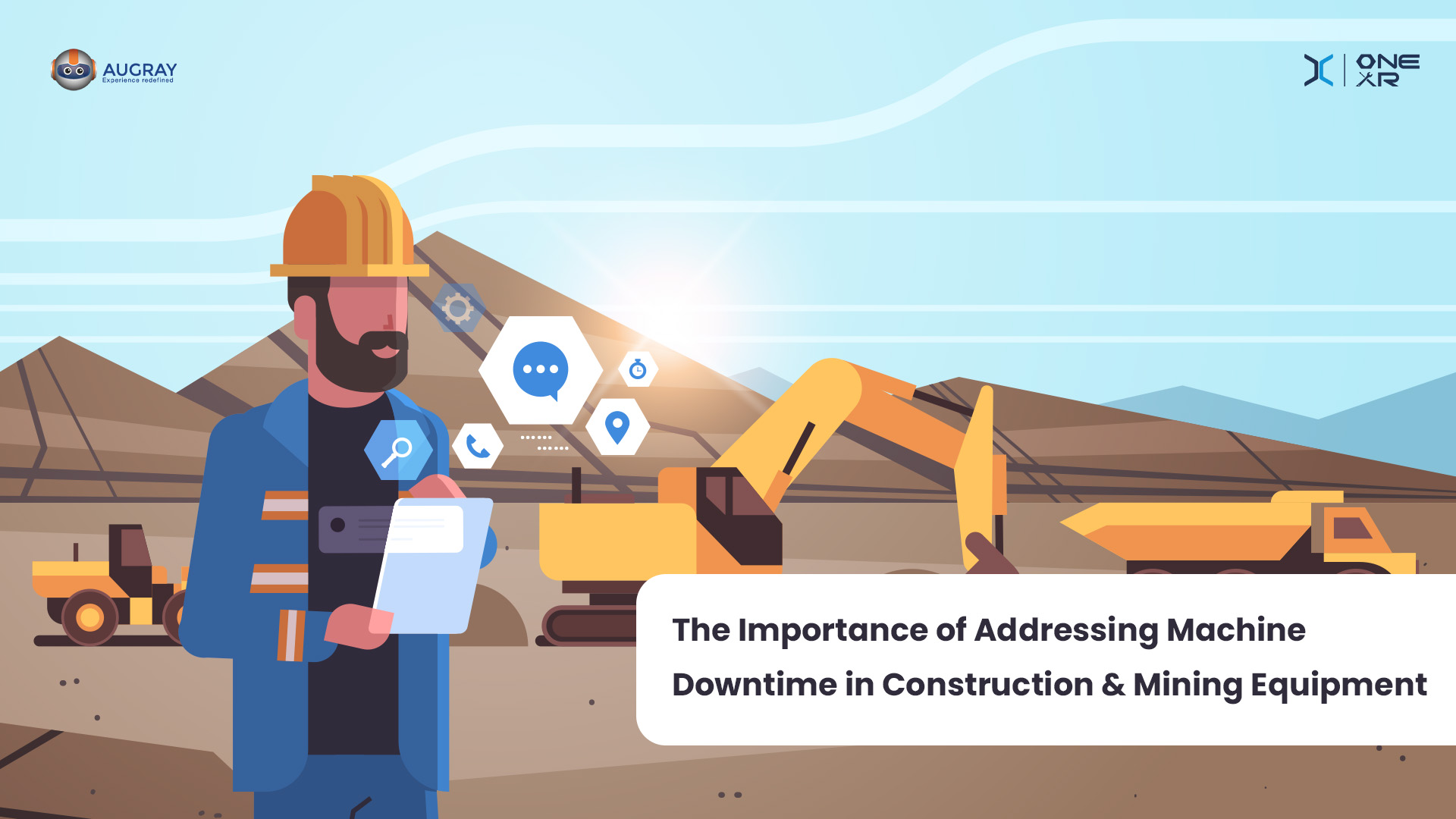The image is an artistic rendition representing the significance of addressing machine downtime and construction in mining equipment, likely designed as the cover page of an article or book. Dominating the foreground, a bearded man with a brown beard and wearing a yellow construction hat stands on a construction site. He is adorned in a blue suit with orange labels and a black T-shirt, suggesting a mix of professional and safety attire. The man holds a clipboard, and around him, various six-sided symbols denote tools like a magnifying glass, a phone handle, a conversation mark, and a location pin, indicating various aspects of jobsite communication and supervision.

The backdrop features a universal brown and tan landscape with a mountain range on the horizon under a sky that transitions from green to blue, with white stripes indicating clouds and a sun partially hidden behind the mountains, casting a distinct light. Three sequences of construction vehicles populate the scene: on the left, a smaller pickup-type vehicle; in the center, a large auger with a crane; and on the right, heavy lifting machinery likely for gravel or mining. The vehicles are painted in shades of yellow, orange, and brown, blending with the earthy tones of the setting.

In the top left of the image is the insignia and brand name "Auger" or "Augury Experience Redefined," while the top right corner bears the brand name "1XR." The bottom right corner features a white box with black text highlighting the core subject: "The importance of addressing machine downtime in construction and mining equipment." This detailed composition uses rich color contrasts and stylized elements to underscore the critical themes in industrial machinery management.